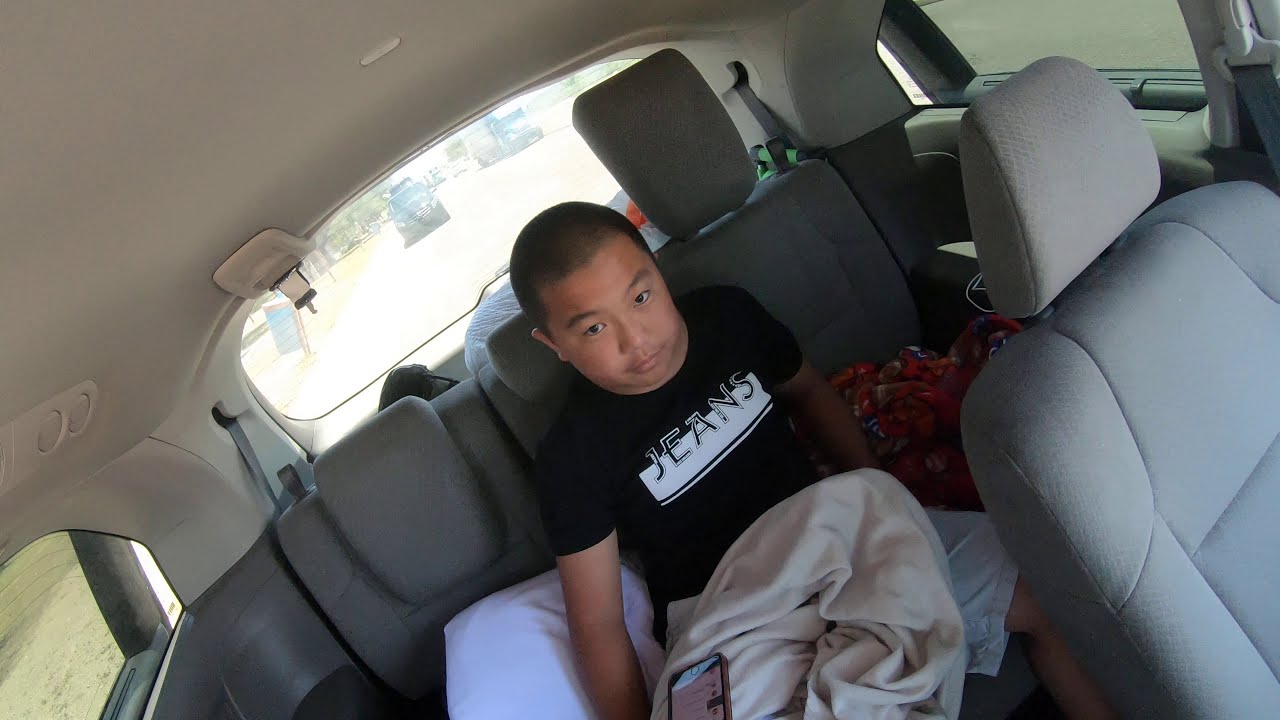The photograph captures a young Asian male with light brown skin, sitting in the middle seat of a car's backseat, appearing slightly tilted to the left due to the diagonal angle of the shot. He has a serious expression on his face, with a buzz cut and a thick neck. The interior of the car features dull, gray canvas seats and a beige ceiling. The male is wearing a black t-shirt with "G-J-E-A-N-S" printed in white over a horizontal white rectangle, and white shorts with a cream-colored blanket on his lap. A smartphone is resting on his right thigh, and a white pillow is positioned next to his right arm. The photograph, taken from the front passenger seat, also captures sunlight streaming through the car’s back window, revealing additional parked cars. The whole scene suggests a calm moment, possibly during a long journey.